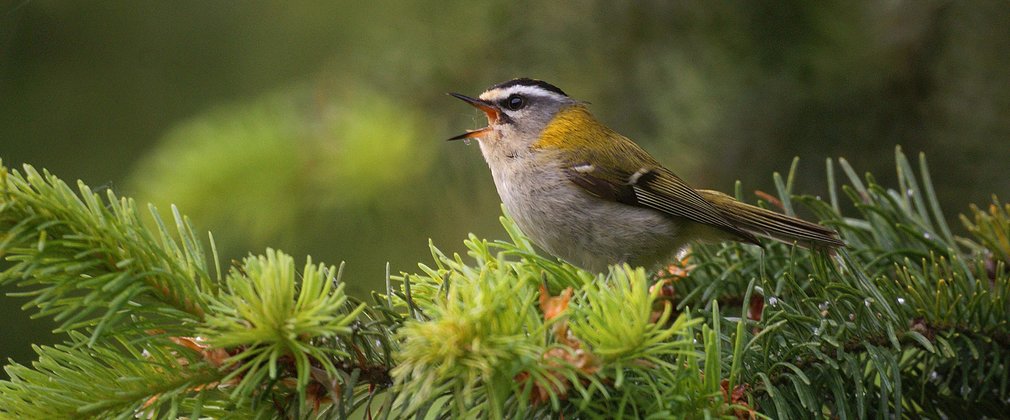This detailed image captures a small bird perched on the branches of an evergreen tree, amidst the vibrant, varied greens of nature. Prominently positioned on a fir tree branch, which showcases both light green new growth and darker, mature needles, the bird is caught in a moment of animated chirping, its beak open wide. The bird's breast is white, transitioning to a mix of yellow and brown on its wings, with the wing tips exhibiting distinctive white stripes. Its head is predominantly grey, accentuated by a striking black stripe running across the top and encircling its eyes. The vivid orange interior of its open beak adds a pop of color to the scene. The background, a tapestry of blurred green hues, suggests the dense foliage of surrounding trees, keeping the focus sharply on the bird. This meticulous capture vividly portrays the essence of the bird's natural habitat, highlighting the intricate details of its plumage and the rich textures of the evergreen branches.